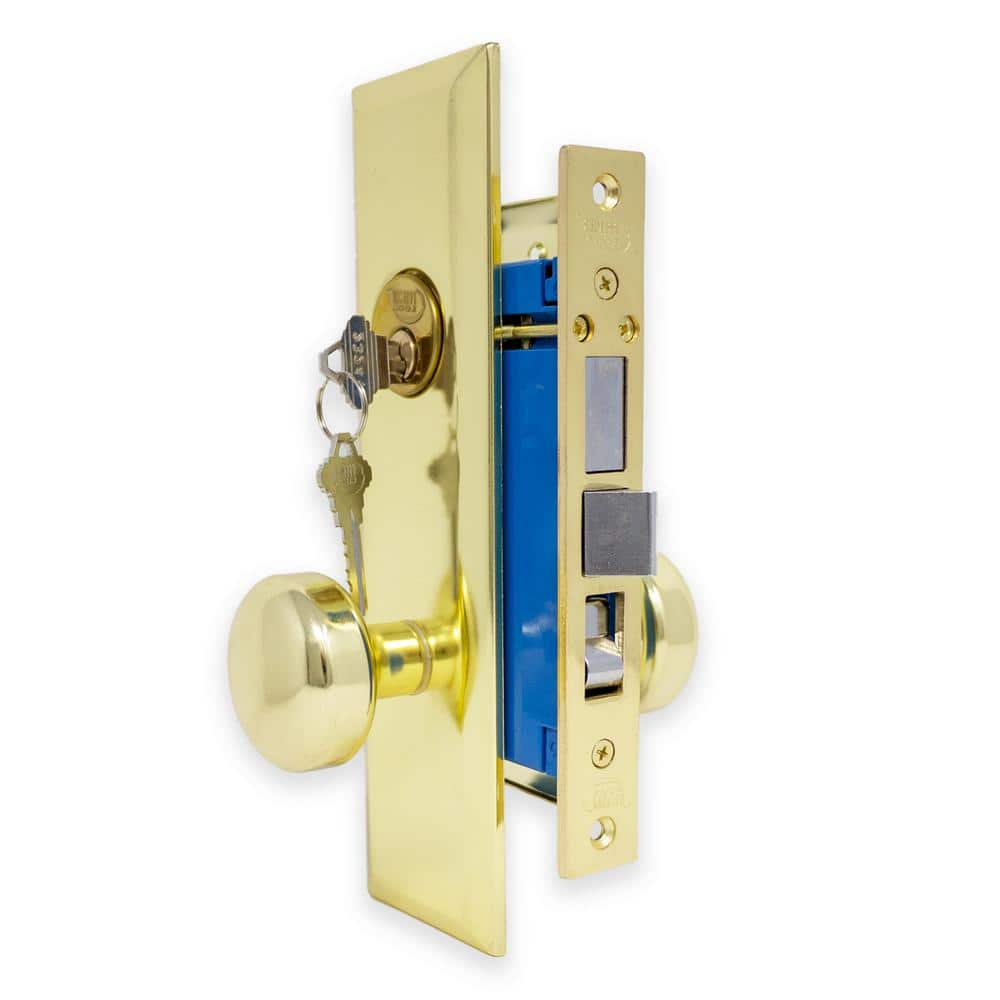The photograph captures a detailed, close-up view of a brass lock assembly, illustrating its various components in an "exploded" view, set against a pure white background. Highlighting both the exterior aesthetic and internal mechanics, the image reveals a cylindrical brass lock plate featuring a double lock system—a non-keyed smooth brass doorknob at the bottom and a keyed deadbolt cylinder at the top. 

A key, brass-colored and distinctive in a sledge shape, is inserted into the deadbolt cylinder, while a matching spare key dangles from a stainless steel split key ring. The mechanism within the lock, exposed to show the internal workings, is characterized by dark blue components, visible screws, and various latching parts made of nickel or stainless steel. The image offers dimensions and forms, suggesting the brass plate to be about five inches high and an inch wide, designed to fit into a door cutout.

This comprehensive depiction emphasizes the lock's shiny brass finish and the dual functionality of the deadbolt and doorknob, intended for enhancing security. The photograph provides not merely an aesthetic appreciation but also an instructive glance at the lock's assembly, underscoring the intricacies involved in installing or replacing a door lock.